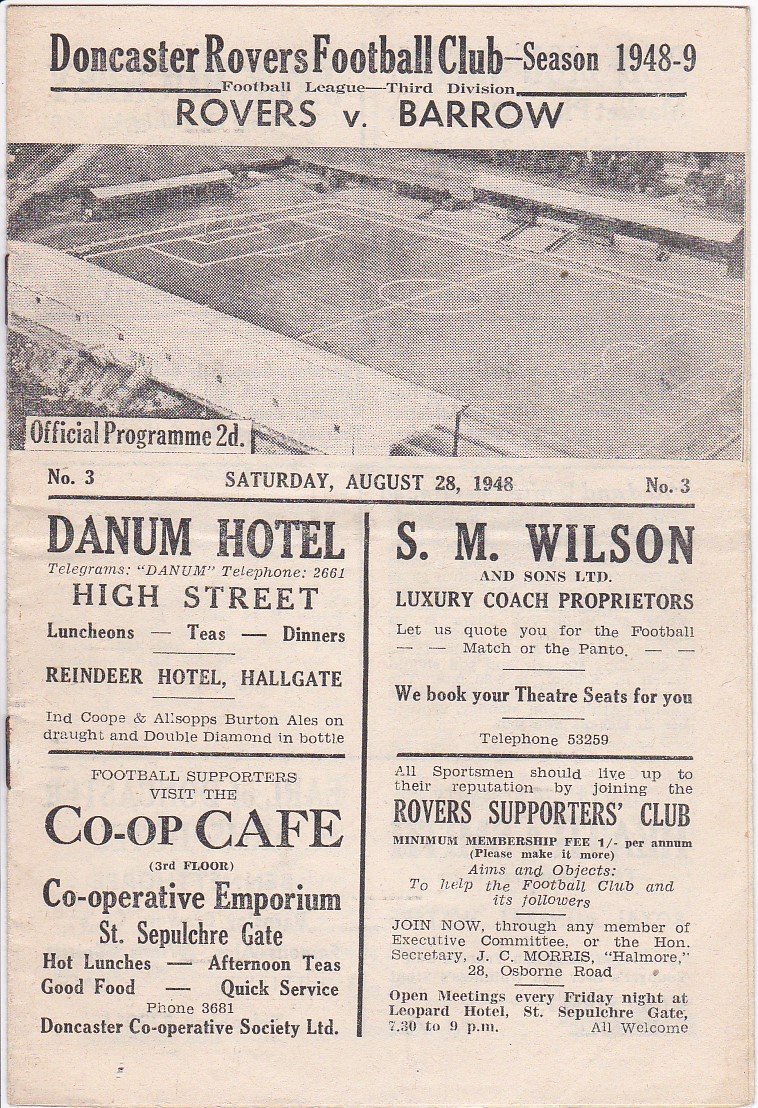This is an image of an official program for the Doncaster Rovers Football Club from the 1948-1949 season, specifically for a match in the Football League Third Division between the Rovers and Barrow. The top of the program is adorned with bold black text stating "Doncaster Rovers Football Club Season 1948-9 Football League Third Division Rovers vs. Barrow." The whole cover is printed in black and white.

At the center of the page, there is a photograph of an empty soccer field, taken from a 45-degree angle starting from the lower-right and extending towards the upper-left. The field is fully marked and ready for play, surrounded by a large but empty stadium. Below the image, the text reads "Official Program 2d" on the left and "Number 3 Saturday, August 28th, 1948" on the right.

The lower section of the program features four advertisements. On the left is an ad for Danum Hotel on High Street with details including "Telegrams: Danum Hotel," "Telephone: 2661," and offerings such as "Luncheons, Teas, Dinners." S.M. Wilson and Sons Limited, Luxury Coach Proprietors, also have an advertisement with a pitch to let them quote for football matches or theater bookings, along with a telephone number "53259."

The bottom ads include one for Co-op Cafe at the Cooperative Emporium, St. Sepulchre Gate, offering hot lunches, afternoon teas, good food, and quick service with phone number "3681." Another ad is for the Rovers Supporters Club, encouraging sportsmen to join with a minimum fee of 1 per annum to support the club and its followers, with meetings every Friday night at the Leopard Hotel, St. Sepulchre Gate, from 7:30 to 9:00 p.m., welcoming all attendees. Contact information provided includes the Honorable Secretary, J.C. Morris, at 28 Osborne Road.